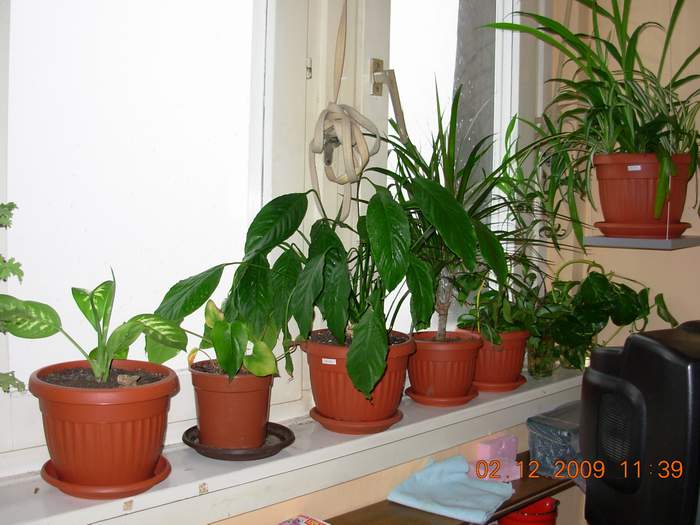This photograph, dated February 12, 2009, at 11:39 p.m., captures a serene indoor scene featuring several potted plants on a white shelf, which is part of a counter cabinet display. The plants, housed in matching terracotta red-orange planters with water catch bowls, appear lush and green, some with visible blooming flowers. They sit by a large window with white shades that allow sunlight to pour in, illuminating the vibrant foliage. In the foreground, a bulky black object is visible, partly obscuring another terracotta pot resting on it. Beneath the window, a blue cloth covers a wooden table, adding a touch of color contrast. To the right, a different type of plant resides in a rectangular reddish planter, contributing to the diverse yet harmonious botanical display. The timestamp and date in orange at the bottom of the photo authenticate this peaceful moment.